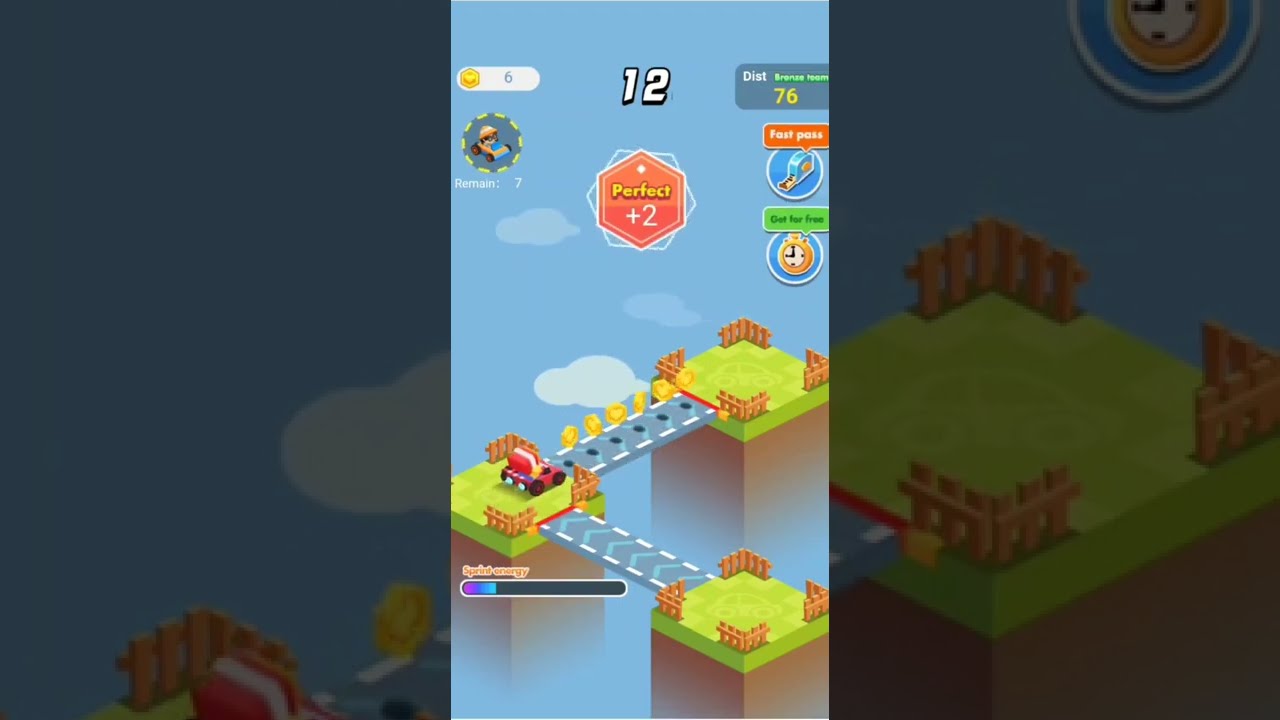This image is a vertical screenshot of a mobile platformer game, captured from a phone. The central focus is on a vibrant, grassy platform landscape dotted with brown fences and interconnected by concrete-like highway bridges, marked with white stripes and blue arrow designs. At the top of the screen, various navigational icons and game stats are displayed: "12" in white at the top middle indicating a timer, "6 remaining" in yellow hexagons on the upper left, and "76" in yellow on the upper right. There's also a pink or orange hexagon bearing the text "Perfect +2." The primary scene features a red car or truck with a flaming exhaust and a red box on its roof, poised on one of the green, grass-topped islands. This vehicle is about to cross a bridge with floating coins ahead, against a backdrop of a blue sky dotted with clouds. The image also includes darkened, enlarged versions of the scene on either side, emphasizing the central gameplay screen.